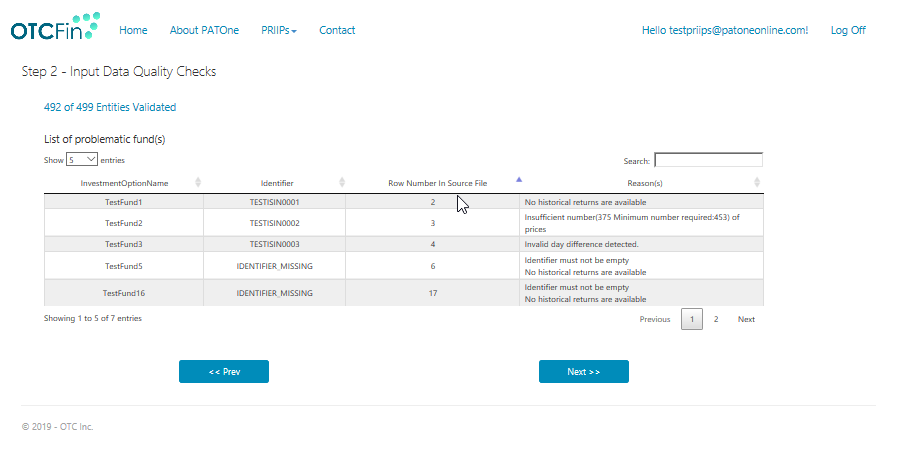A detailed caption for the image could be:
---
The image displays a computer screen dominated by a blue interface from a software named "OTCFIN." At the forefront, there is a "Step 2: Input Data Quality Checks" section, which includes a list of test funds labeled Test Fund 1, 2, 3, 5, and 16. In the text, it shows validation information indicating that 492 out of 499 entities have been validated. The rows and columns resemble a table, possibly from a database interface rather than a traditional Excel file. The visible part of the table lists row numbers and source files 2, 3, 4, 6, and 7. A prominent horizontal menu bar at the top includes tabs labeled "Home," "About," "PAT1," "PRIPS," "Contact," and more. Additionally, an active cursor is positioned over the first entry, highlighting Test Fund 1 with an ISIN (International Securities Identification Number) of 0001. Other text on the screen includes "Hello Test Prep Set" and "pat1online.com," suggesting this is part of a financial data validation or management system.